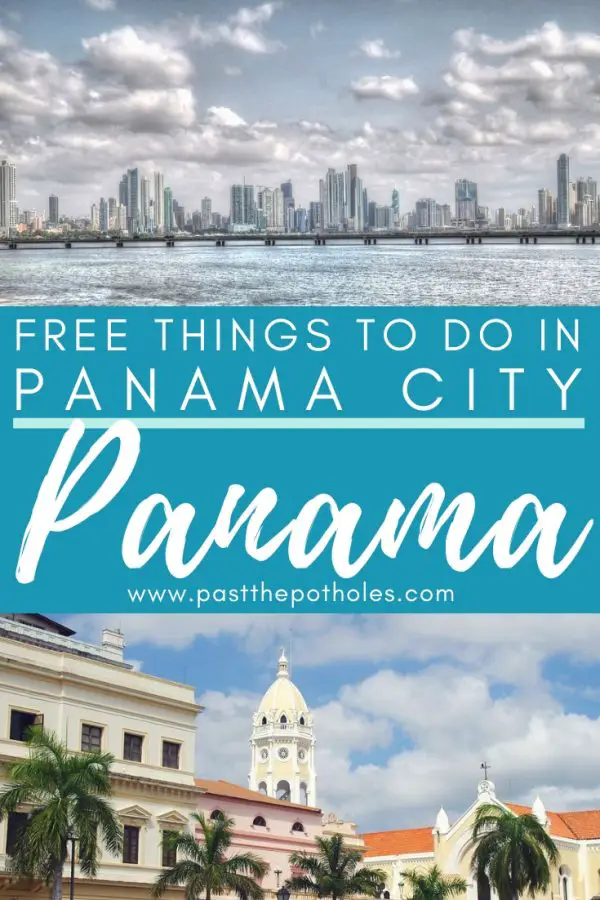The brochure titled "Three Things to Do in Panama City, Panama" features vivid imagery and detailed suggestions for visitors. Dominating the center of the design is the main title, accompanied by the URL "pastthepotholes.com."

The upper section displays a stunning photograph of Panama City's downtown skyline. The horizon is peppered with numerous tall buildings beneath a partly cloudy sky. In the foreground, a prominent bridge stretches across the frame, offering an intriguing perspective of the city's infrastructure.

Beneath this, the bottom section presents an image capturing the charm of the local architecture. A notable edifice, possibly a historic church or city hall, stands out with its yellowish paint, dome, and reddish-orange roof. Adjacent to it, there is a smaller, possibly two- or three-story building that resembles an office.

Overall, the brochure suggests several cost-free activities in Panama City, Panama, highlighting both its modern skyline and rich architectural heritage.